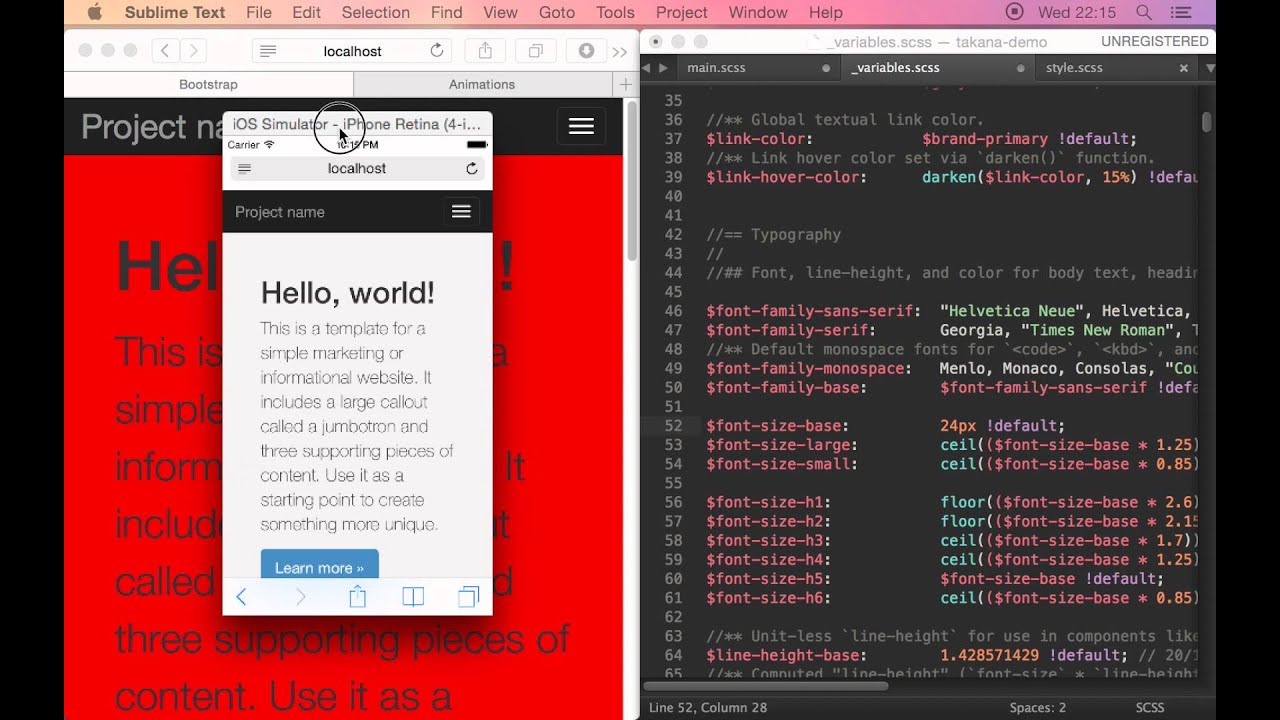The image displays a split-screen browser window. On the left side, there is a website with a red background and black text titled "Hello World" at the top. The page features a description about the template beneath the title, while in the upper left corner, there is a note mentioning a project. The address bar indicates that this website is being hosted locally, as it shows "localhost". Additionally, a pop-up window is visible, stating "iOS Simulator iPhone Retina 4". At the bottom of the webpage, there is a prominent "Learn More" button, which is blue with white text.

On the right side of the screen, there is a coding or settings panel displayed against a black background. The panel showcases lines of code numbered from 35 to 65. The code is color-coded with various hues including red, black, purple, orange, green, and a yellowish-orange, indicating different elements and syntax in the code.